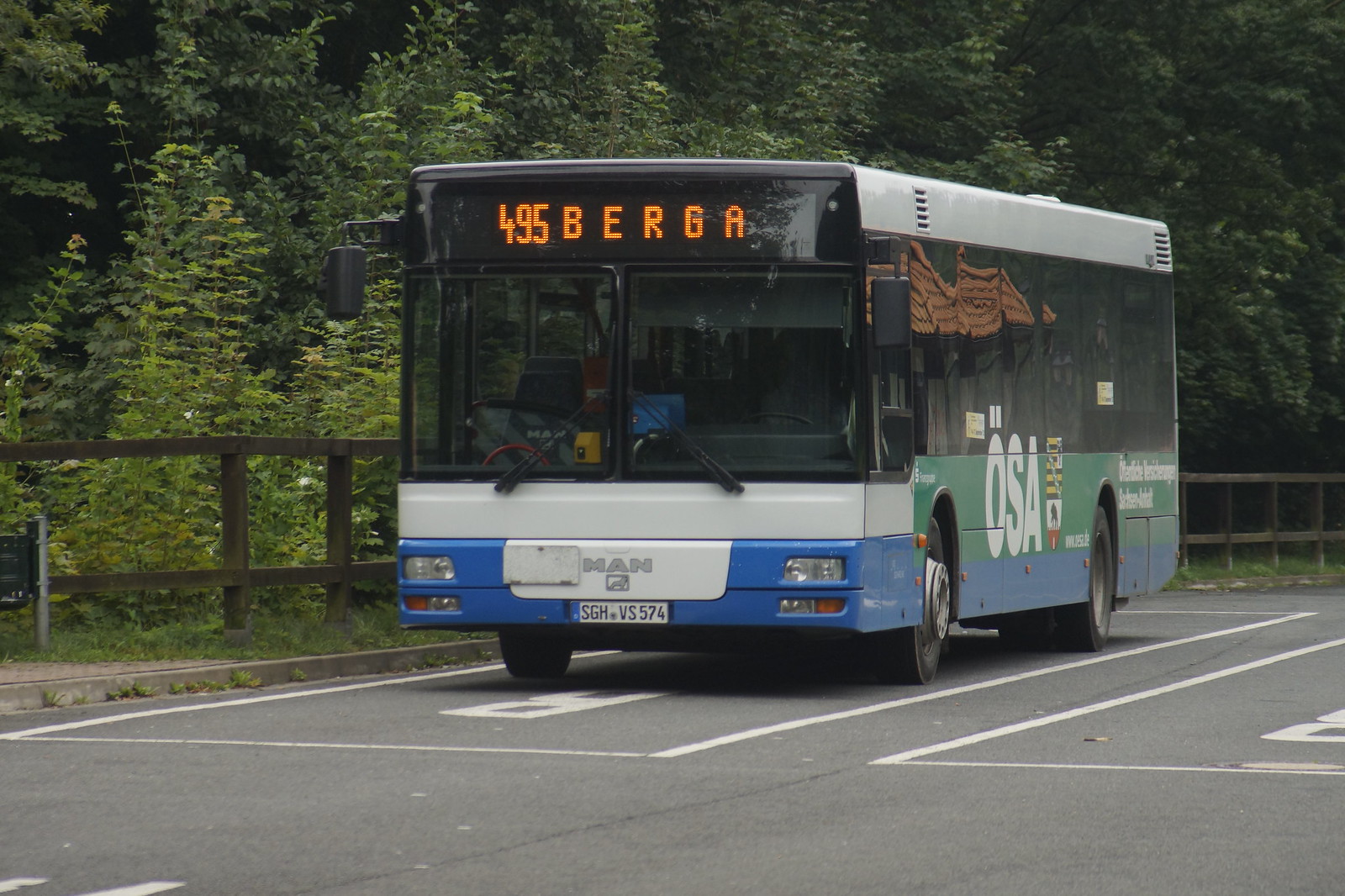This detailed photograph captures a European bus, stationary in a clearly marked parking spot on a gray asphalt lot. The bus, predominantly blue and white with green and black accents, prominently displays an illuminated sign reading "495 Berga" in orange letters. Below the windshield, a blue bumper is bisected by a narrow white stripe, which features the manufacturer name "MAN" in the center. The windshield has two large panes separated by a black strip, with wipers converging at the midpoint. Moving down the side, the bus includes silver trim at the top, windows stretching about half its length, and a green stripe above the blue bottom trim. The side also bears the letters "OSA" and an undiscernible white text near the rear. Beyond the bus, a brown wooden post rail fence runs parallel and is backdropped by a dense forest extending across the entire scene. The absence of a visible driver confirms the bus is parked, with no people in sight.